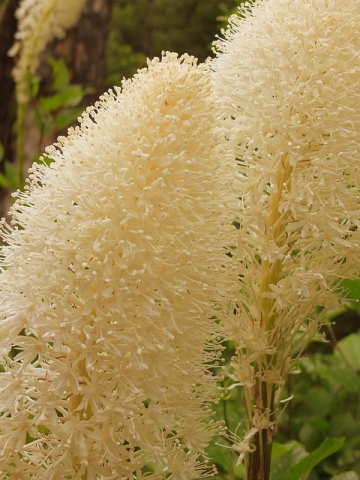In this professionally taken photograph, two large, cone-shaped clusters of countless off-white, creamy beige flowers dominate the composition. The flowers, consisting of smaller florets grouped together to form a larger inflorescence, are meticulously captured in sharp focus, highlighting the intricate details and the soft, almost luminescent quality of the petals. The foremost flower extends from the bottom left nearly to the top, while a slightly taller cluster appears behind it on the right. The background is gently blurred, accentuating the focal flowers and creating a dreamy, ethereal effect. Subtle hues of green and brown, along with hints of reddish tones and taupe, provide a serene backdrop with what appear to be green leaves and a tree trunk emerging on the top left. The overall scene suggests an outdoor setting, possibly in a forest or garden. The ambient light enhances the natural beauty of the flowers, making them stand out against the subdued, leafy background.